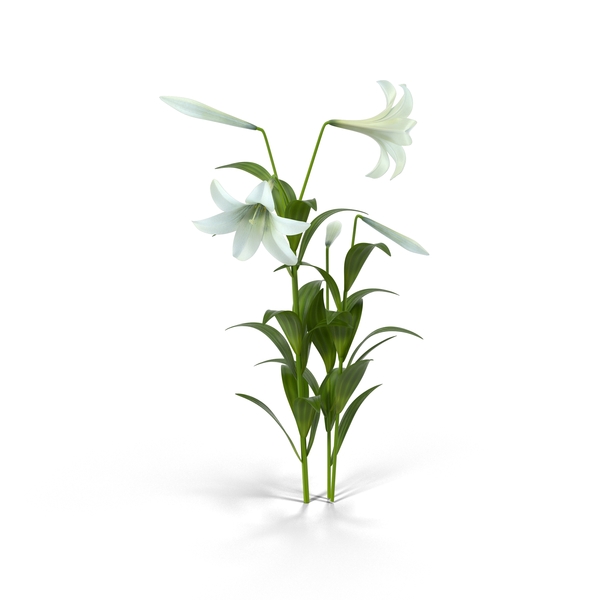The image showcases a stark white background with three green stems bearing white lilies. Two of the stems are prominent and situated closely together, while the third is slightly hidden behind them. Each of the stems is adorned with lush green leaves. There are a total of five leaves on the primary stem, and each of the secondary stems also carries a set of leaves, making an approximate count of around twenty leaves in total. Among the blooms, there are two fully opened lilies, each displaying their six large, prominent petals. Additionally, there are three unopened lily buds present on the stems. The open blooms face different directions, adding a dynamic feel to the composition, which with its pure white background, emphasizes the delicate beauty of the white lilies and the contrasting greenery.